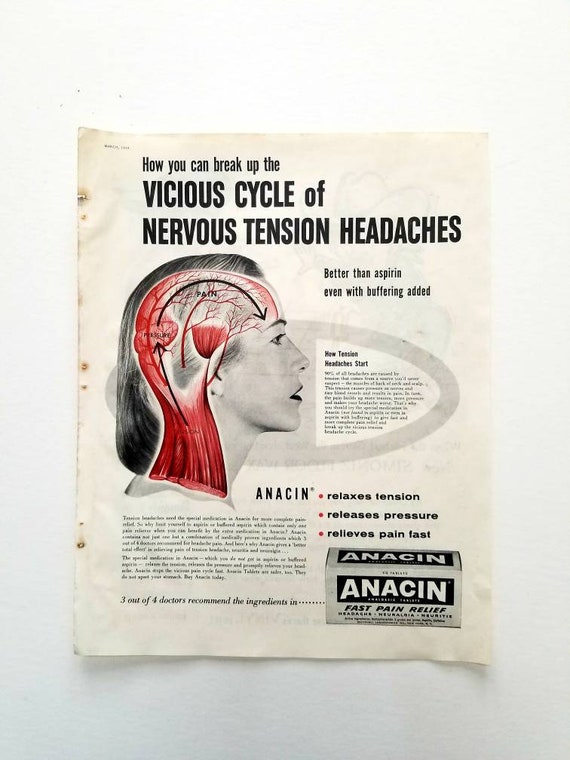This image is a photograph of a slightly yellowed and somewhat deteriorated page, likely torn out of an old magazine from the 70s or 80s. The page features an advertisement titled in bold black print, "How You Can Break Up the Vicious Cycle of Nervous Tension Headaches." Below this headline, it emphasizes Anacin's superior efficacy, stating, "Better than aspirin, even with buffering added."

Dominating the center of the page is a black and white profile image of a woman facing right. Overlaid on her head are detailed illustrations of the neural network and neck muscles, highlighted in red, with black arrows pointing from her neck to her forehead, illustrating the origin and path of tension headaches.

To the right of her image, a snippet of text begins with "How tension headaches start," although the full paragraph is too small to read clearly. Further, aligned to the right, another bold text asserts, "Relaxes tension, releases pressure, relieves pain fast," adjacent to an illustration of an old-style Anacin box marked "Fast Pain Relief."

At the very bottom of the page, it declares, "3 out of 4 doctors recommend the ingredients in Anacin," underscoring its medical endorsement. The ad is primarily monochromatic, save for the red accents on the illustration, reinforcing the clinical, informational tone of the advertisement.